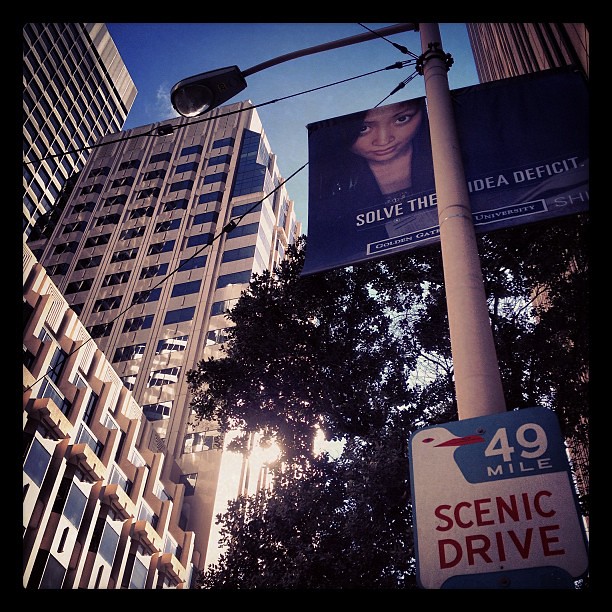The image captures an urban scene from a low vantage point, looking up at towering skyscrapers in a downtown setting. Dominating the foreground is a white lamppost extending towards the top center of the picture. The lamppost is adorned with two distinct signs. The lower sign is blue, featuring the text "49 Mile" and a red arrow pointing left, with an illustrated seagull above the words "Scenic Drive" on a white background. Above this, there is a black canvas banner displaying an image of a woman, accompanied by the words "Solve the Idea Deficit." This banner is partially obscured by the lamppost, suggesting it could be an advertisement, possibly for a university. The surrounding buildings are modern and tan-colored with dark-tinted windows, and a prominent white building, approximately 20 to 30 stories high with numerous windows, stands to the left. The sky above is clear and blue, with sunlight illuminating the scene.